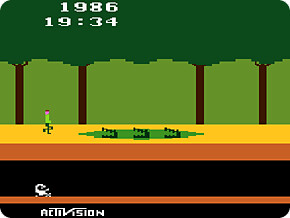The image is a colorful screenshot from a vintage video game. At the top of the rounded rectangular frame, it prominently displays "1986" in white font, alongside a digital time reading "19:34." The background features a lush landscape populated with trees. In the foreground, a small character is seen walking on a vibrant yellow platform. Below this platform is a green pond, depicted with open-mouthed alligators that seem to be waiting below. An orange line separates this scene from a thick black border, under which rests a small, unclear white image on an orange platform. At the very bottom, another black line frames the image and bears the text "Activision" in white, indicating the game's publisher.